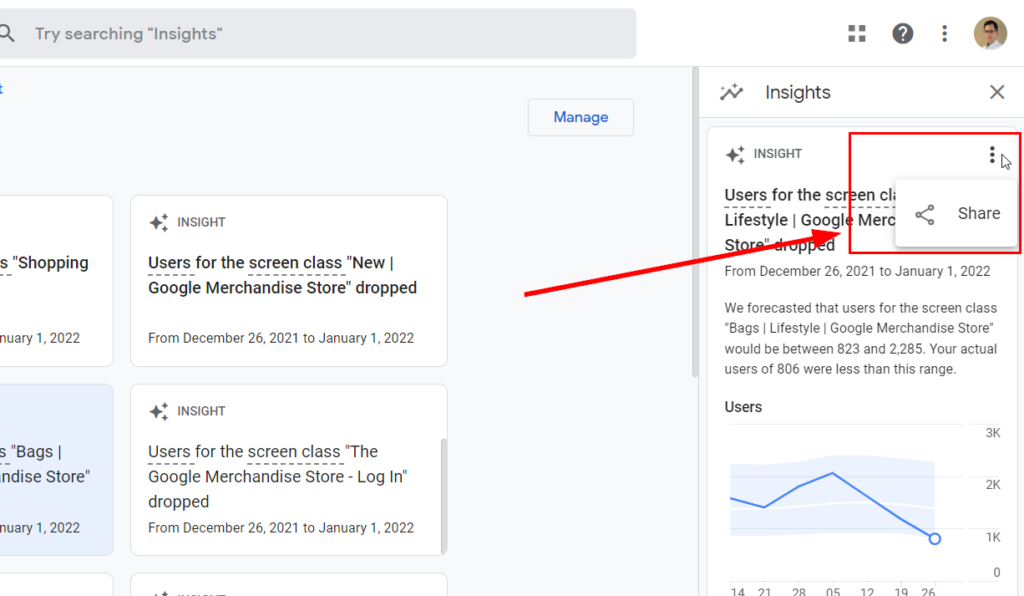Screenshot Caption: Detailed View of Web Development Analytics Platform

This image is a detailed screenshot from what appears to be a web development analytics platform, displaying various insights and data points related to user interactions. The interface features a predominantly minimalist design, with black text on a white background.

In the upper left-hand corner, there is a search bar with the placeholder text “Try searching insights”. The right-hand side of the top bar contains several icons: four small squares, a question mark, three vertical dots, and a circular profile image of a Caucasian individual wearing a white top.

The left panel has a dark grey background and displays sections separated by rectangles. The text within some of these sections is only partially visible. The visible text includes two insights:
1. "Insight: Users for screen class 'new Google merchandise store' dropped from December 18, 2021, to January 1, 2022."
2. "Insight: Users for screen class 'Google merchandise store login' dropped from December 28, 2021, to January 1, 2022."

There is also a blue "Manage" button at the top right corner of this section.

The right panel is a white background that begins with the header "Insights". Below this header, there appears to be a repetition of the first piece of insight text from the left panel. A red arrow points from the first insight text box on the left panel to the right panel, indicating an area of focus. Additionally, a red square covers a "Share" button, perhaps highlighting an important feature.

Further down, more detailed information about the analytical insights is presented. It forecasts that users for the screen class "Bags lifestyle Google merchandise store" will range between 83 and 286. The actual user count is indicated to be 886 or fewer within this range. Following this, there is a section labeled "Users" accompanied by a graph showing a reduction in user numbers over time.